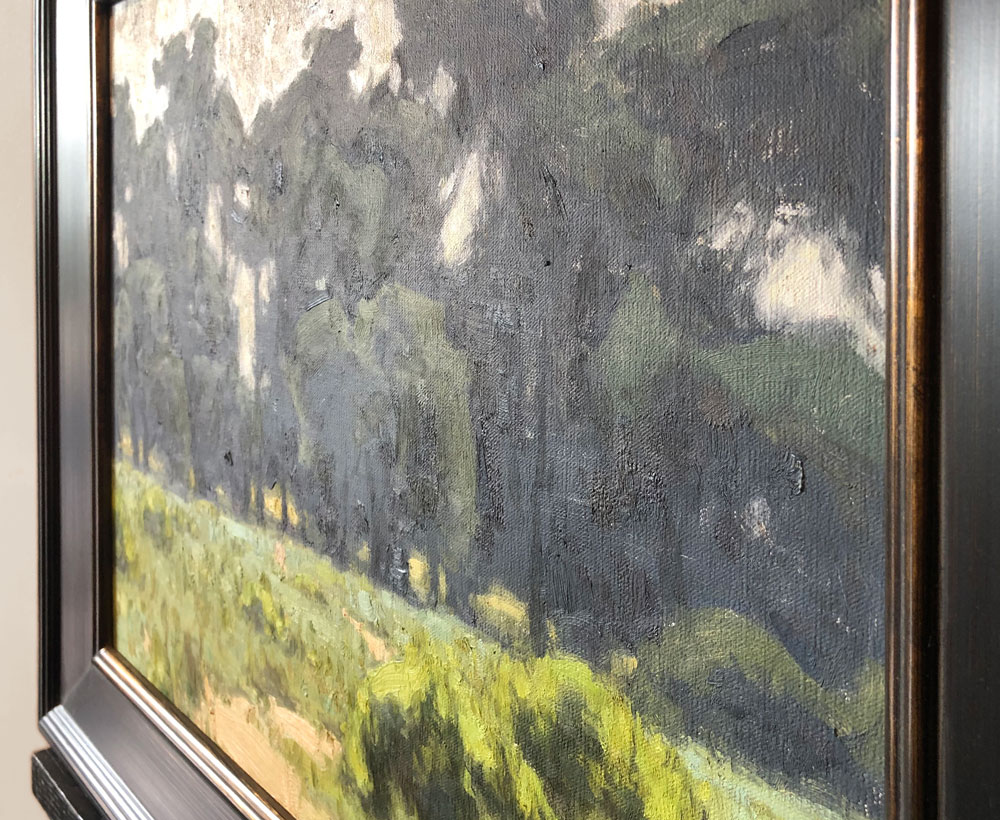The photograph captures a side-angled view of a painting hanging on a wall, allowing only a partial view of the artwork. The painting is encased in a wide, dark brown wooden frame with subtle gold accents, and it's situated on a black shelf. The scene within the painting portrays an outdoor landscape, featuring a vibrant, green grassy foreground interspersed with patches of brown soil. On the right side of the painting, there is a vivid green bush. Beyond the grassy area, a stand of trees with dark forest green foliage rises in varying heights. Above this arboreal setting, a light gray to pinkish-cream sky extends across the top of the artwork, creating a serene atmospheric effect. The photograph’s steep angle reveals the depth and texture of the painting, giving a dynamic perspective from the right side, looking towards the left.